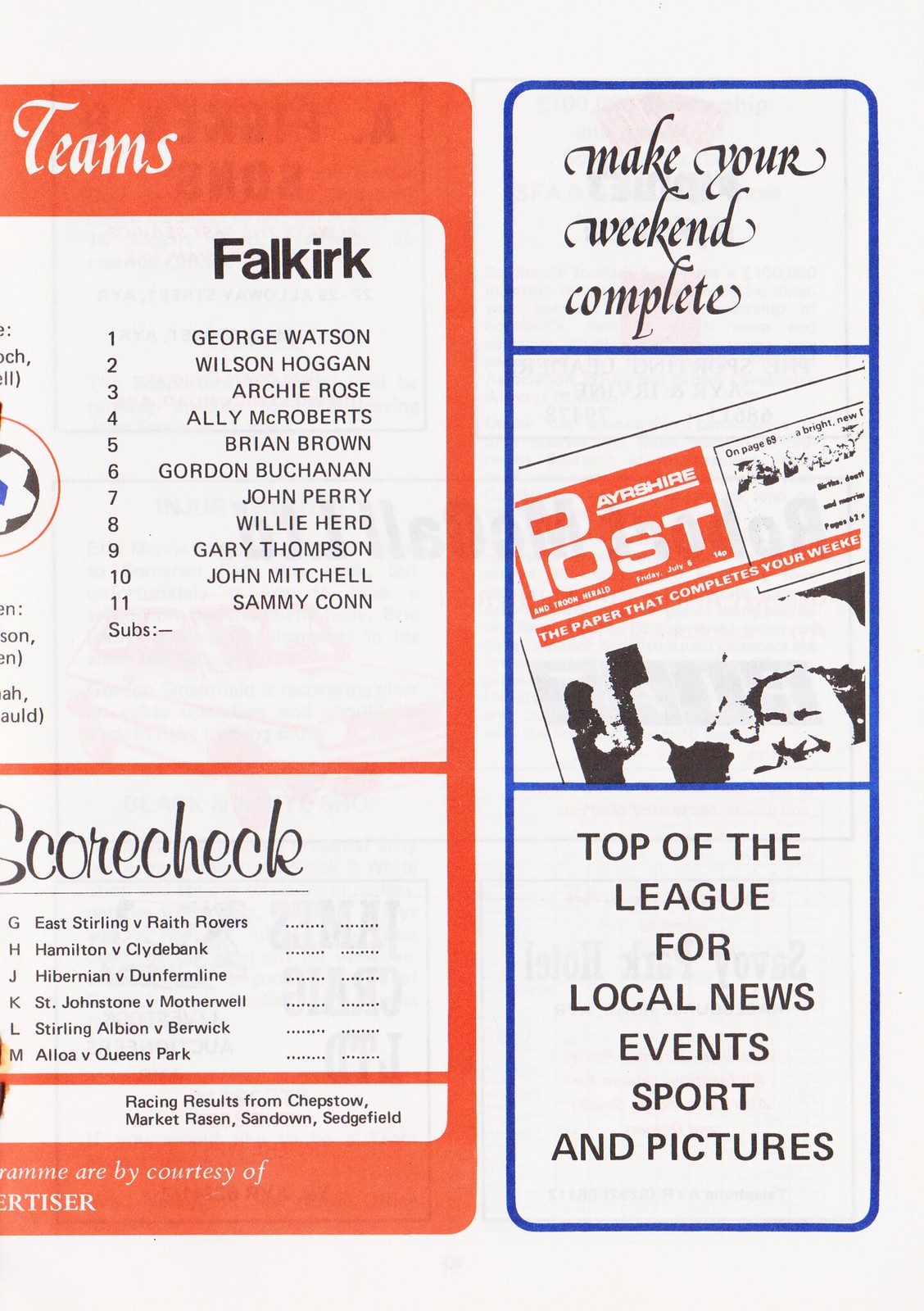The image portrays a vintage-style publication page, divided into two distinct vertical sections. The left section, partially cut off, features an orange border containing black text listing football players under the heading "Falkirk," with names such as George Watson, Wilson Hagen, Archie Rose, Allie McRoberts, and more. The top of this section is marked by a red box with white text reading "teams," and the bottom portion is devoted to a "scorecheck" area for noting scores next to team combinations. The right section, outlined in blue, promotes the Ayrshire Post, featuring black text that invites readers to "Make Your Weekend Complete." This advertisement highlights the newspaper's offerings—local news, events, sports, and pictures—touted as "Top of the League." The page presents a glimpse into a vintage football program scorecard, smoothly blending informative content with promotional material.